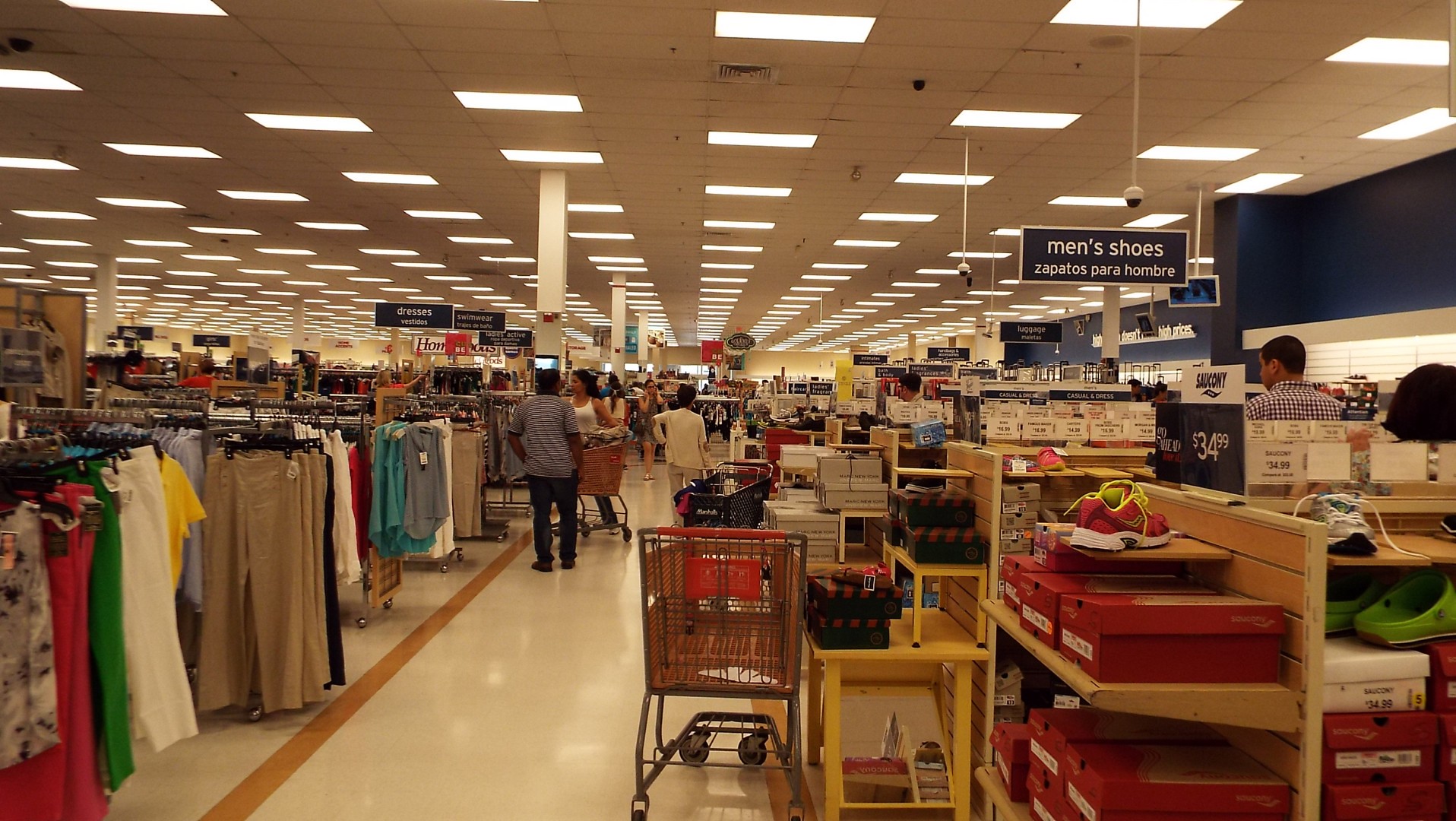The image depicts a department store interior with a central aisle stretching away from the photographer. Two shopping carts, one red and one gray, are positioned in the aisle, and a pair of women with another red cart are shopping nearby. Overhead on the left, a sign with white lettering on a dark background reads, "Men's Shoes, Zapatos para Hombre." Opposite this, on the right-hand side, the wall is blue and lined with shoe racks displaying a variety of footwear including red tennis shoes with yellow laces, white tennis shoes, gray and white shoes, and Crocs. The shoe shelves also contain red shoe boxes. A man wearing a plaid shirt stands with his back to the viewer in the shoe section. On the left side, another overhead sign reads "Dresses, Vestidos," above racks holding women's clothing such as shirts, slacks, and pants, which are organized on black hangers. The store's floor is white with an orange or red stripe, and the ceiling features a grid of rectangular lights illuminating the entire scene.